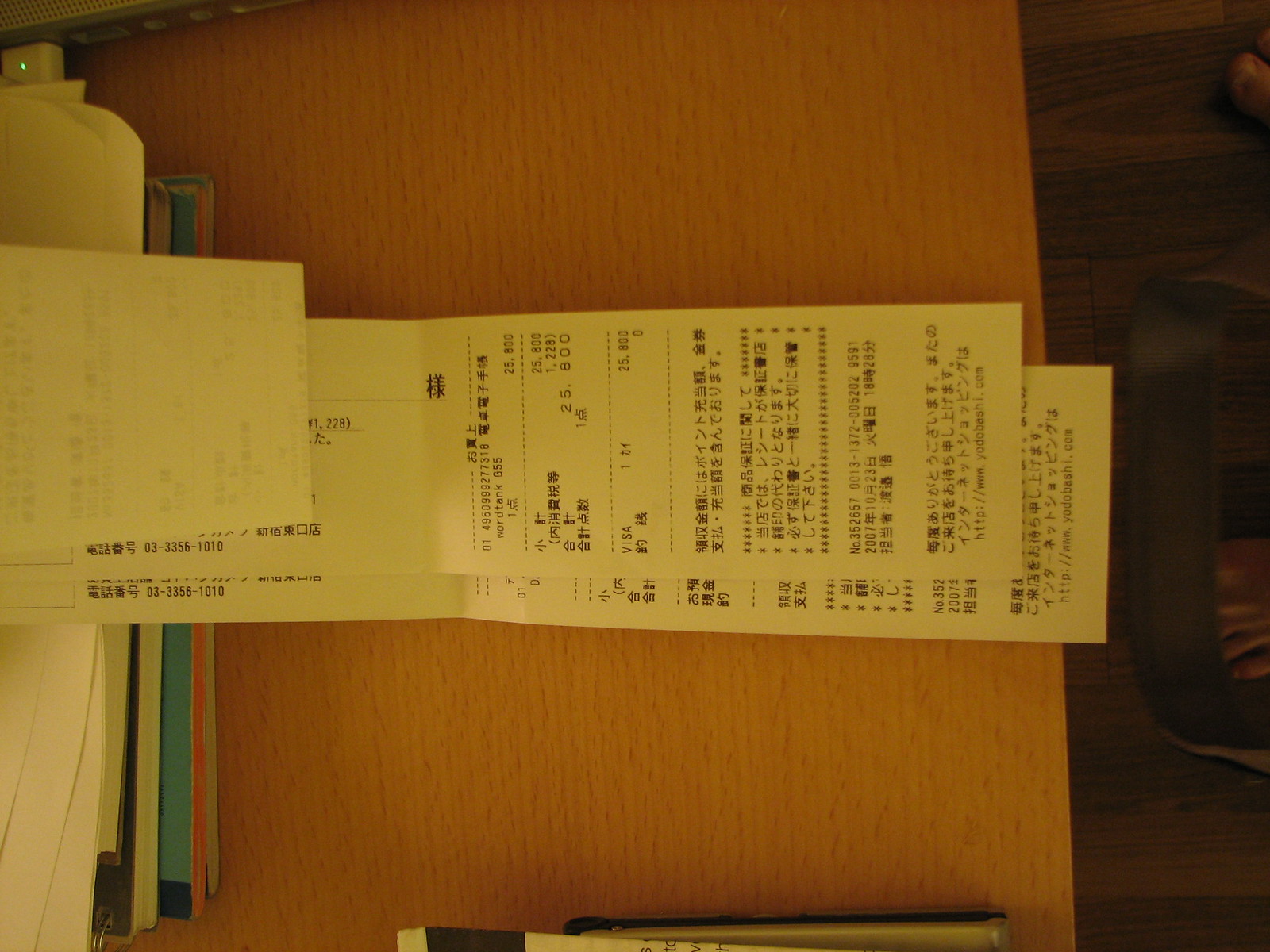This landscape-oriented color photograph captures a scene primarily showcasing two or three receipts, which are laid one on top of the other on a surface that mimics an artificial wood effect. The receipts, displaying traditional Japanese characters, are slightly tilted, necessitating a 90-degree anti-clockwise head turn to read them properly. They appear highly detailed, with black and white text featuring several sections divided by dashed lines, and one of them indicating a price of $25,800 in an unspecified foreign currency. A barcode and possible tracking information suggest they might be related to shipments or postal services.

The wooden surface, with its grain running from top to bottom, has accompanying shadows at the bottom, indicating a dimly lit environment with some reflection from an overhead light. The receipts are partially resting on a stack of varied colored items, including folders and notebooks, positioned slightly off the left edge of the frame. To the right, the desk or table ends, revealing a wooden floor. The darkness and shadows obscure some items at the edge of the table, adding a subtle depth to the photograph.